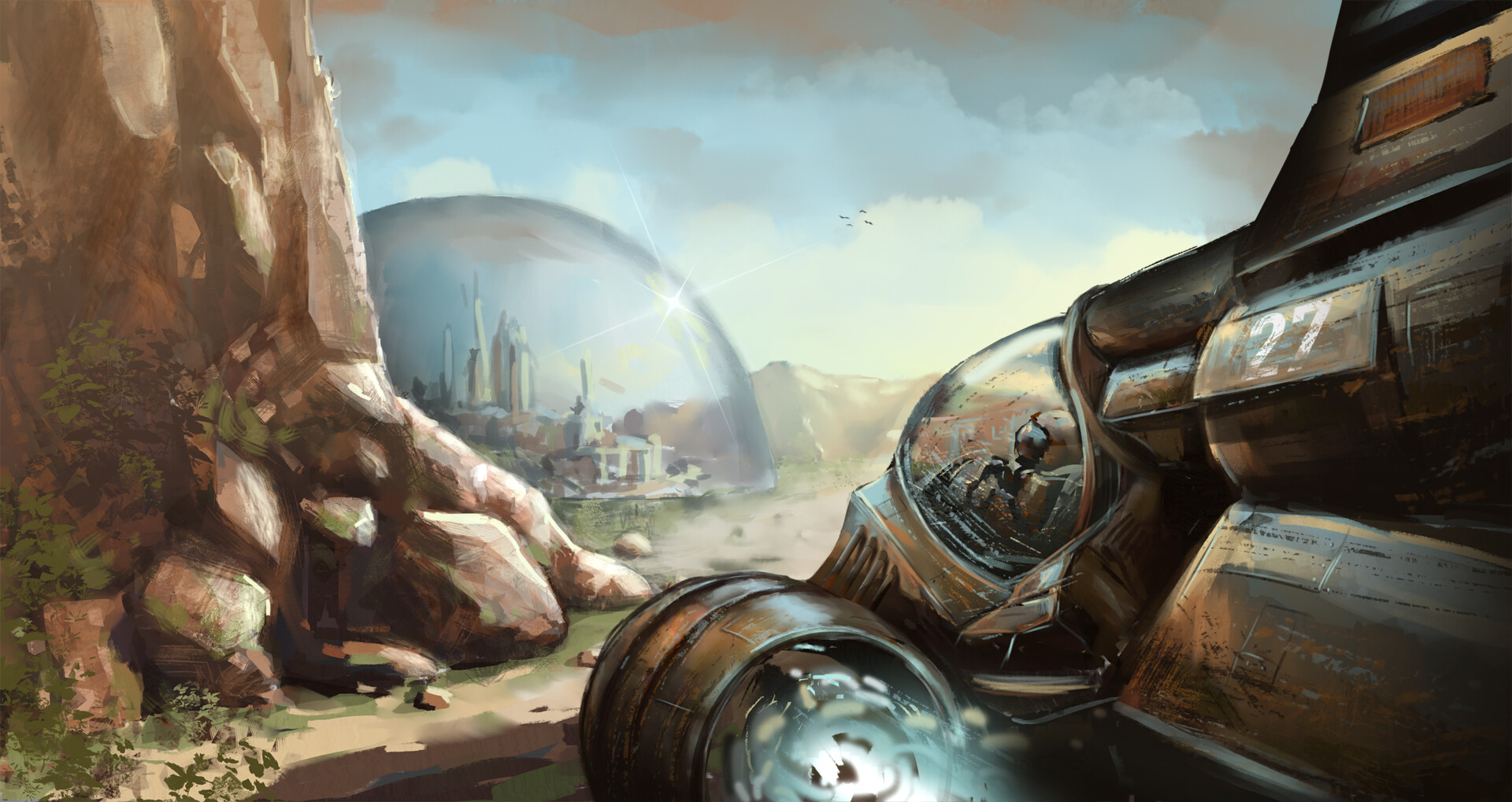This digitally created art piece illustrates a fantastical Martian city on an alien world, evoking a Star Wars-esque storyboard. In the foreground on the right of the image sits a metal brown spaceship with its thruster still on; the spaceship has a glass windshield through which a helmeted astronaut is visible in the control area. Notably, the ship bears the number "27" in white on its side. Surrounding the ship, the ground is comprised of various shades of tan and brown dirt. To the left, the landscape features land and rock formations in differing shades of brown, accented by occasional green leaves. In the far background, a mountain range rises under a sky painted in diverse hues of blue and white. Also in the distance, white buildings resembling a castle sit beneath a protective air dome. Adding life to the scene, small faint black lines, possibly birds, can be seen flying in the sky, enhancing the narrative depth of this bright and clear setting, which is rich in detail and color.